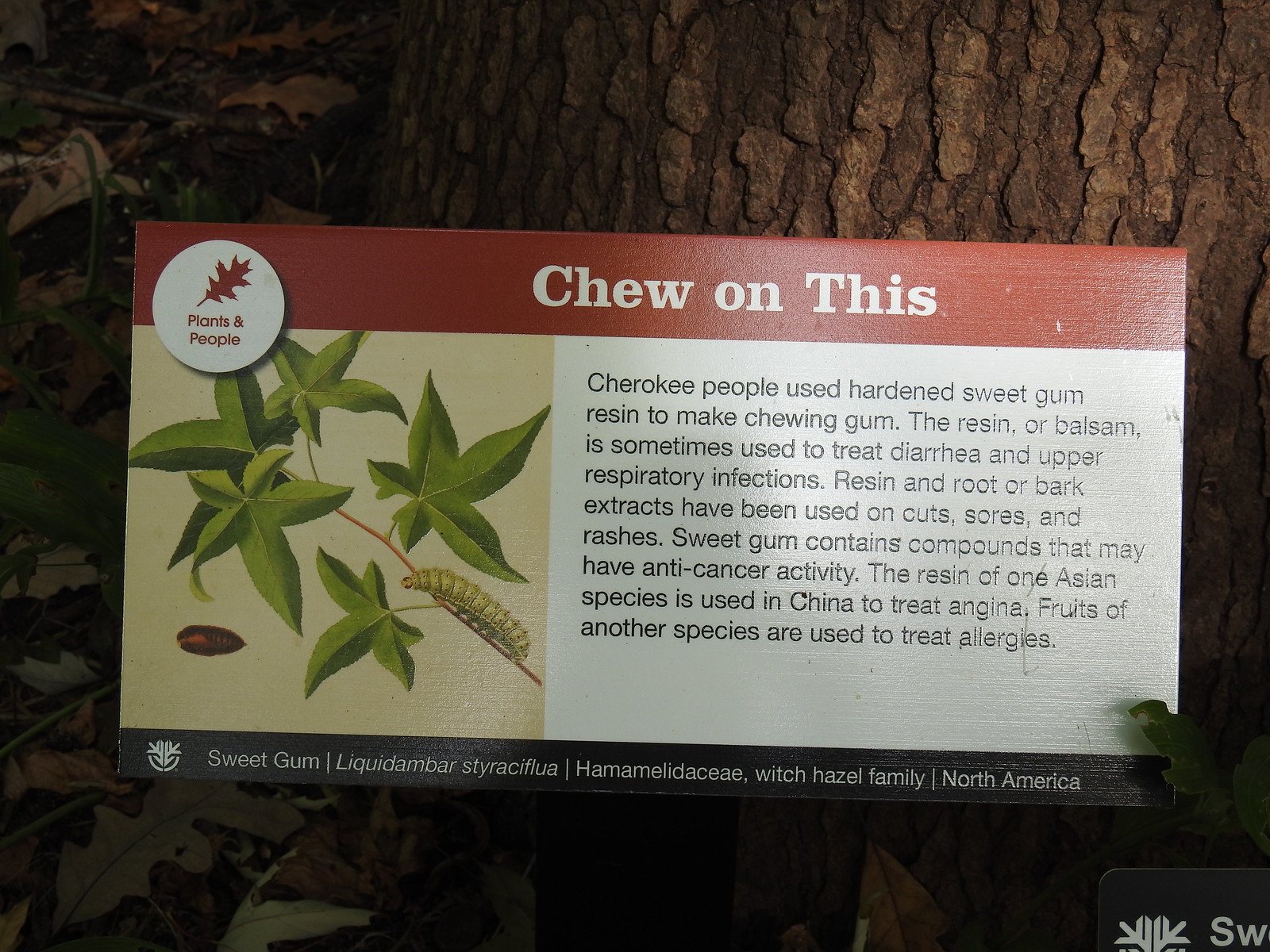The image depicts an informative sign affixed to a tree, possibly within a museum setting. The sign prominently features the heading "Chew on This" in white text at the top. On the left side, within a circular emblem, is the phrase "Plants and People" with an illustration of a red leaf. Below this, a painting of star-shaped leaves, accompanied by a caterpillar on a branch, is shown. The text on the sign details historical and medicinal uses of the sweet gum tree:

- Cherokee people traditionally used hardened sweet gum resin to create chewing gum.
- The resin, also known as balsam, is sometimes utilized to treat diarrhea and upper respiratory infections.
- Extracts from the resin, roots, or bark have applications in treating cuts, sores, and rashes.
- Sweet gum contains compounds with potential anti-cancer properties.
- In China, resin from an Asian species of sweet gum is used to treat angina, and fruits from another species are used to treat allergies.

At the bottom, the sign provides the scientific name of the sweet gum tree, noting that it belongs to the witch hazel family and is native to North America. In the background, a tree and some foliage are visible, complementing the natural theme of the display.